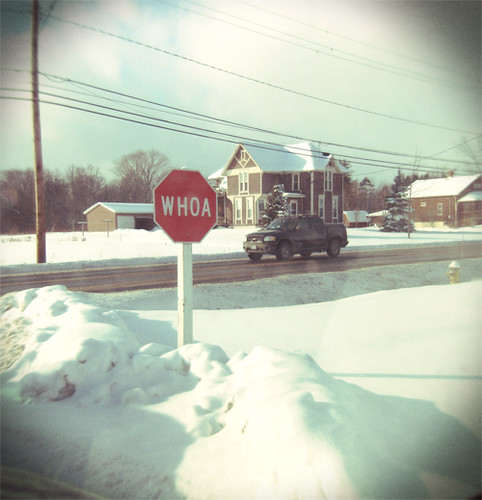This color snapshot depicts a winter scene, likely in North America, showcasing a heavily snow-covered landscape. Central to the image is a modified stop sign, buried in about three feet of snow. The sign, traditional in shape and color, instead bears the word "WHOA" in bold white letters. Positioned slightly left of center, its white post is partially obscured by the surrounding snow. 

In the background, large and small brick houses are visible, their roofs also blanketed with snow. A small brick house with two outhouses stands to the right of the frame. There’s also a notable presence of phone lines and a large telephone pole extending across the scene, adding to the everyday urban setting. To the right, a small fire hydrant is partly buried under the snow.

In the foreground, a black pickup truck is parked on a snow-lined street. The road itself runs roughly horizontally across the scene. The photograph features a gradual vignette, causing the corners to fade into darkness, which draws the viewer’s focus toward the detailed wintry center. In the background, amidst the large brick structures, leafless trees add to the stark, cold atmosphere of the image.